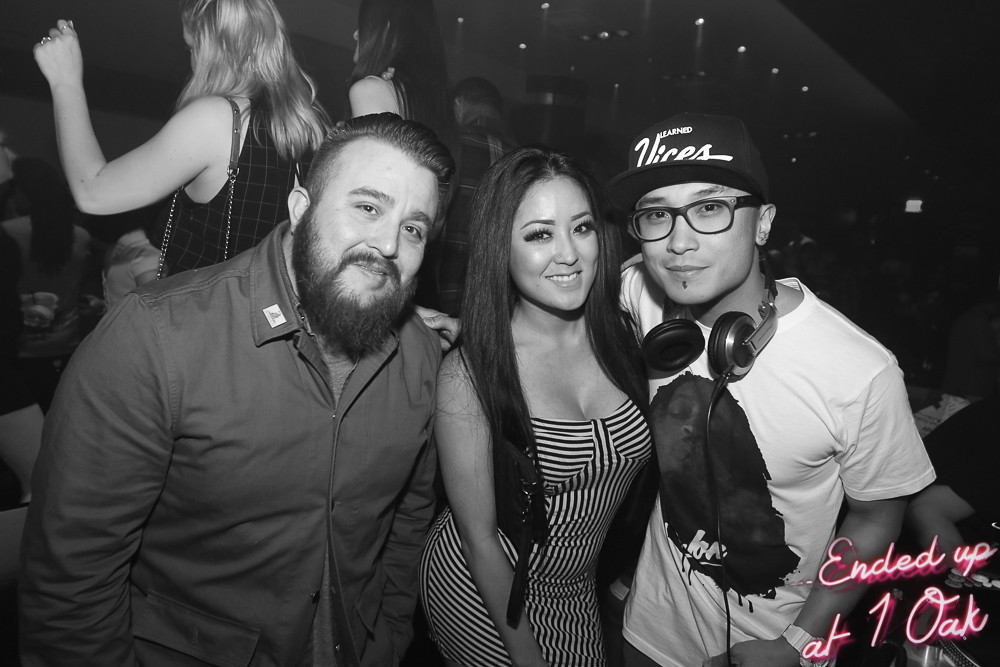In this black-and-white photograph set in a nightclub, three main individuals are prominently featured at the center, posing for the camera. To the left stands a heavyset man with a full beard, short dark hair, and a dark button-up shirt. Next to him, in the center, is a striking woman with long dark straight hair cascading past her chest, dressed in a tight, black-and-white strapless striped dress showcasing ample cleavage. To her right is a young Asian man, wearing a black baseball cap with the words "learned vices" in white, black horn-rimmed glasses, and a white short-sleeved t-shirt with an image of a black man's face on it. He also sports a pair of black headphones around his neck, hinting at his role as the DJ. In the background, lively partygoers can be seen dancing. Directly behind the man with the beard is a young woman with blonde hair, one hand raised and the other holding a purse on her shoulder, wearing a black top. Another woman, facing away from the camera with long brown hair and a plaid dress, is also dancing nearby. Above them, scattered lights or possibly mirrors contribute to the vibrant atmosphere of the scene. At the lower right corner of the image, the phrase "Ended up at One Oak" is stylishly inscribed in a scripted, neon pink font.